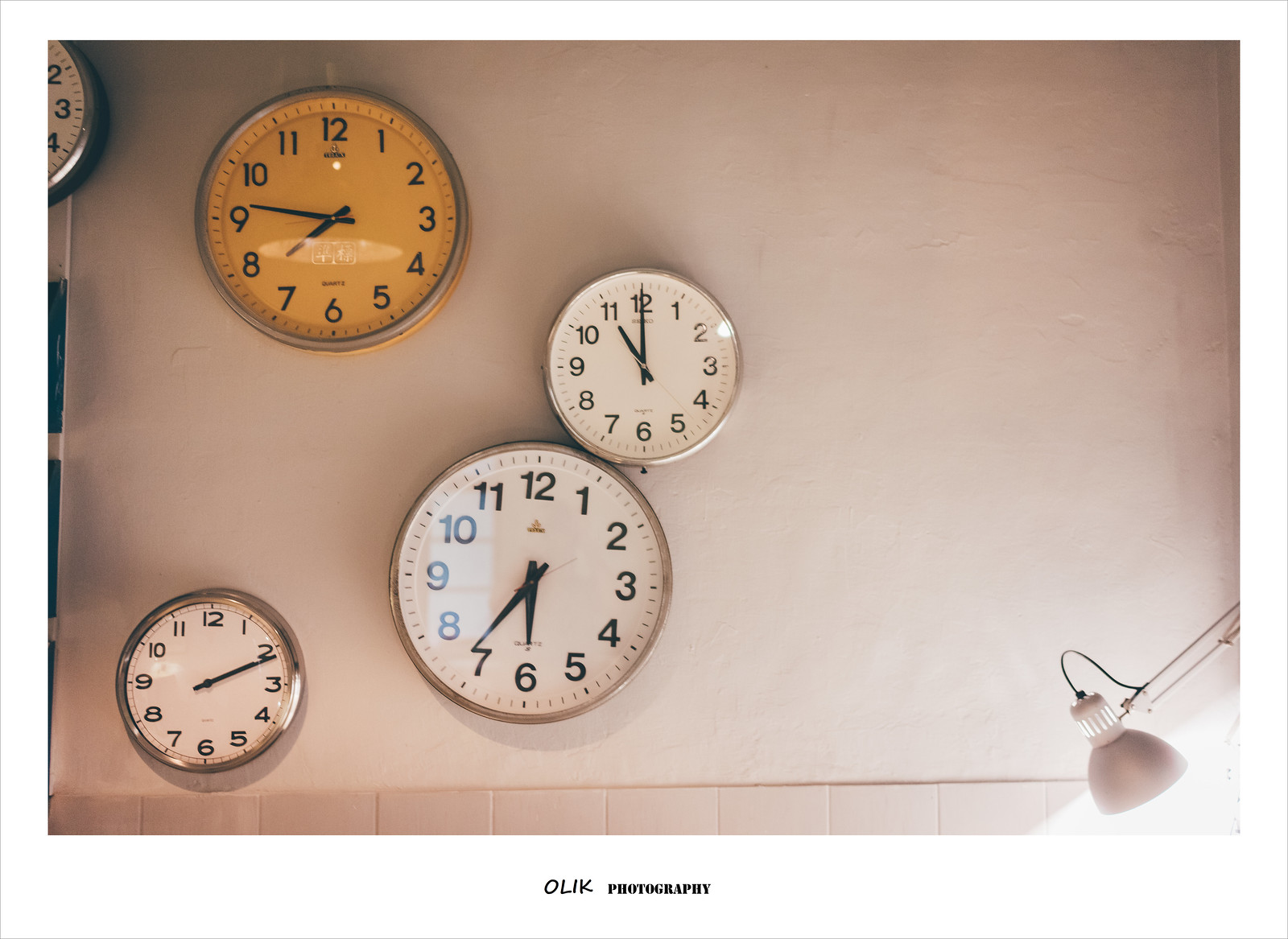The image depicts a wall adorned with at least five round clocks of varying sizes, each encased in either glass or clear plastic. All clocks feature black numerals and black hands on a primarily white background, creating a stark contrast. Notably, the top clock in the center stands out with its vivid yellow face, diverging from the monochrome theme. The yellow clock bears the word "Quartz" prominently on its face. Two of the clocks have additional inscriptions just below the 12 o'clock position, although the exact text remains illegible. The entire display is mounted against a whitish-beige backdrop, enhancing the visual appeal of the uniform but distinct array of timepieces.